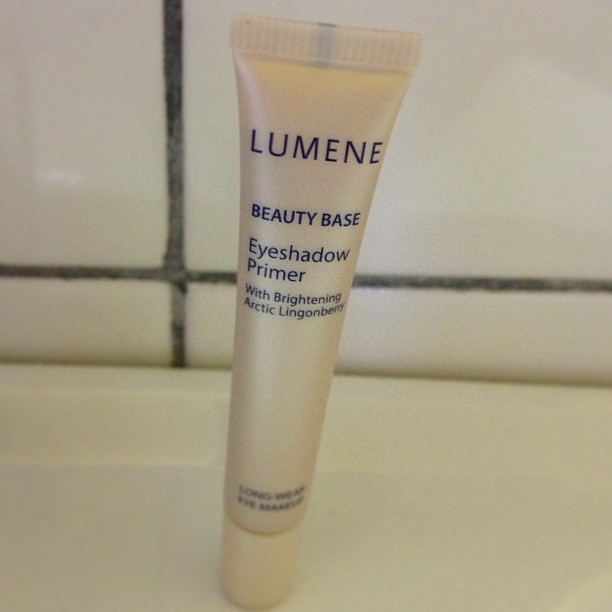The image depicts a slender, off-white to pearl-colored tube of eyeshadow primer resting on a glossy, off-white porcelain surface, likely the top of a toilet lid or a sink. The tube features dark text in uppercase letters: "LUMENE" at the top, followed by "BEAUTY BASE," "EYESHADOW PRIMER with BRIGHTENING ARCTIC LINGONBERRY," and "LONGWEAR EYE MAKEUP" towards the bottom. The cap is frilled and ridged, matching the tube's color. The background consists of shiny white tiles with gray and black grout lines, suggesting it is set in a bathroom. The image is dimly lit, making the tube's color appear grayish in the poor lighting.